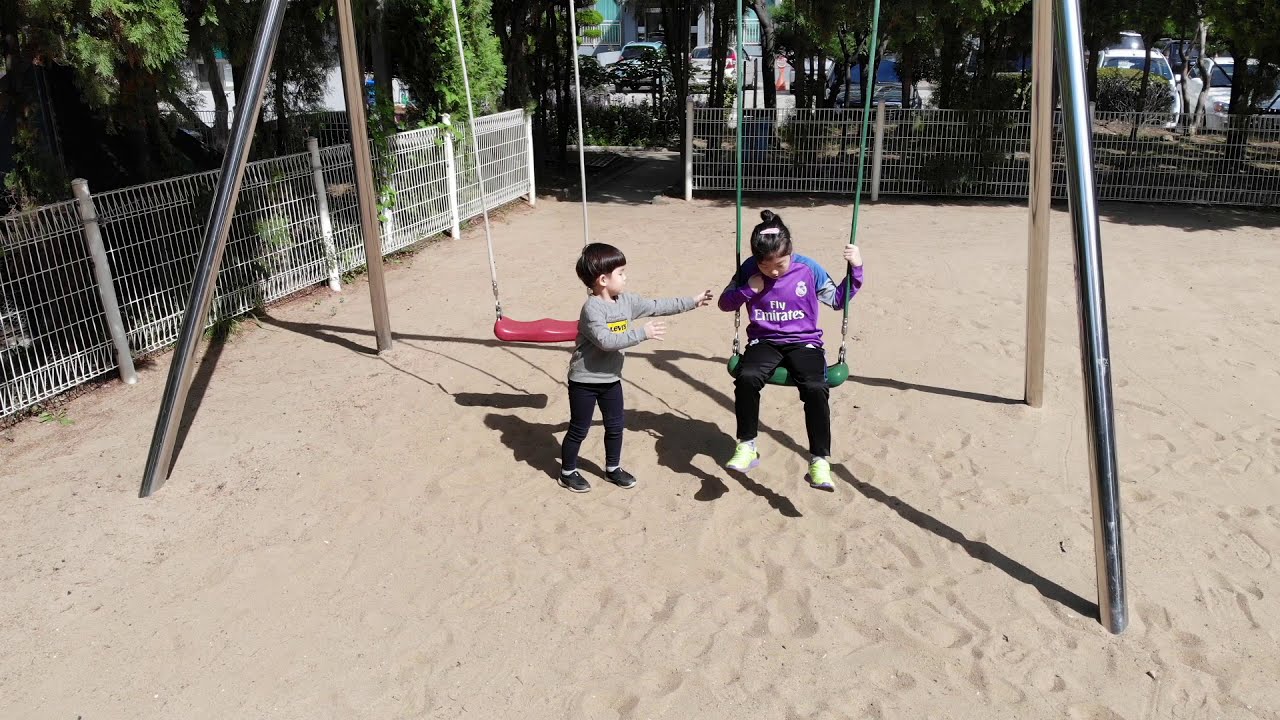In this photograph, two children of Asian descent are at a playground, playing on a swing set enclosed by a white metal fence. The ground is covered in sand. The girl, appearing to be slightly chunky, sits on a green swing with her head bent downwards. She is dressed in a purple, long-sleeved "Fly Emirates" t-shirt with white lettering on the front and black pants. Her dark hair is styled in a ponytail and bun. She is wearing light green and white shoes, and she holds onto one of the swing's lines with her hand while her other arm is wrapped around the swing, her hand resting underneath her chin. To her left, there is a boy, approximately 6 or 7 years old, standing by a red swing. He has short dark hair and is reaching out towards the girl with his arms outstretched. He is wearing a gray long-sleeved t-shirt with a small, indistinct yellow emblem on the chest, black pants, and black shoes. Behind the swing set, thick green trees cast dark shadows, and beyond the trees, some cars are visible, indicating a nearby parking lot.